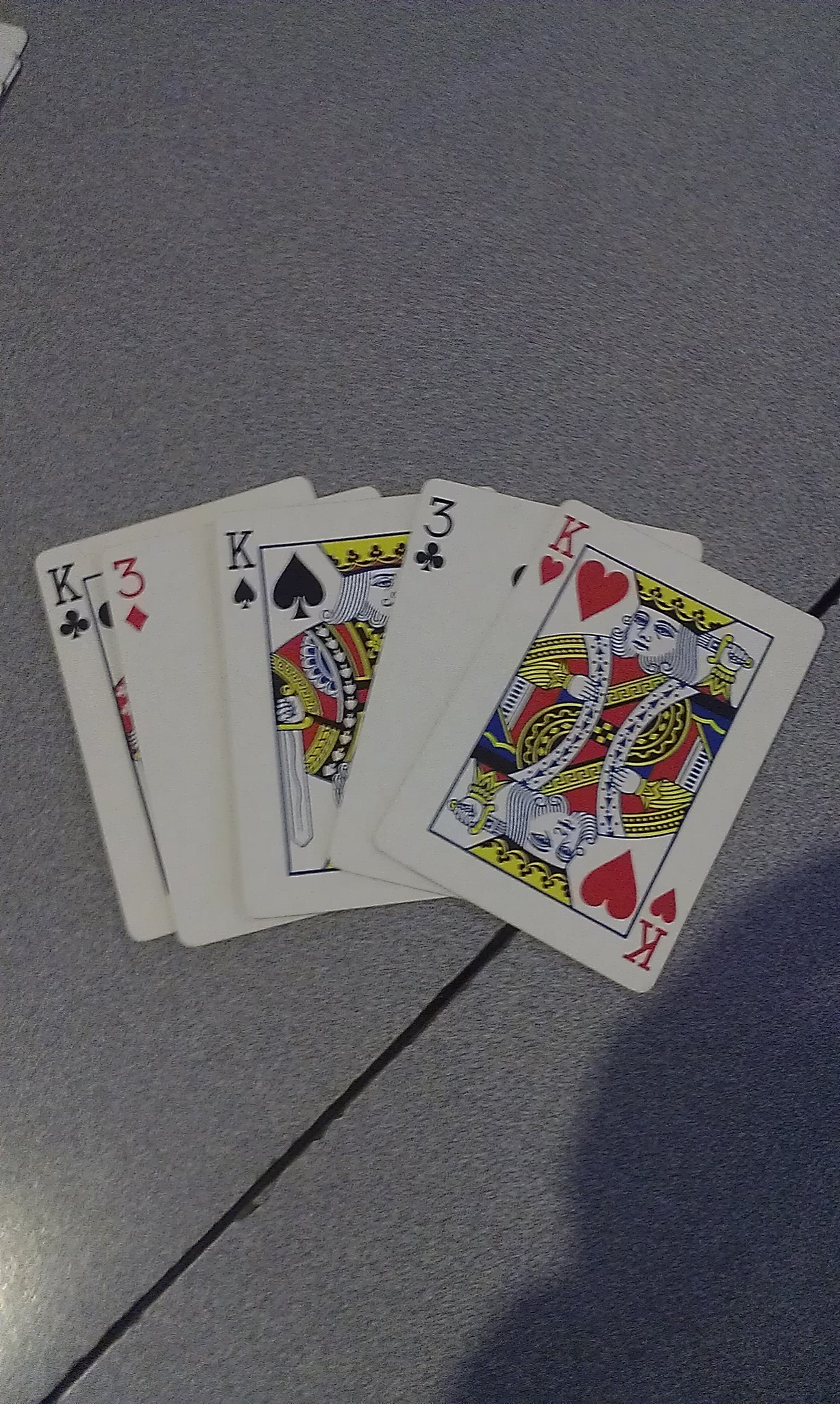A color photograph captures a hand of playing cards lying on what appears to be a concrete surface, with a noticeable relief gap between slabs suggesting an outdoor setting. The lighting indicates a sunny environment, with distinct sunlight and shadow patterns visible on the gray background. The cards are slightly fanned out and include, from left to right, a King of Clubs, a Three of Diamonds, a King of Spades, a Three of Clubs, and a King of Hearts—illustrating a specific combination in poker involving only kings and threes. In the lower right corner, a large, bumpy shadow hints at a person's presence, while the lower left corner shows part of a glowing orb, likely a reflection from a light source. A tiny white protrusion appears in the top left corner, possibly the corner of another card, though its identity remains unclear.